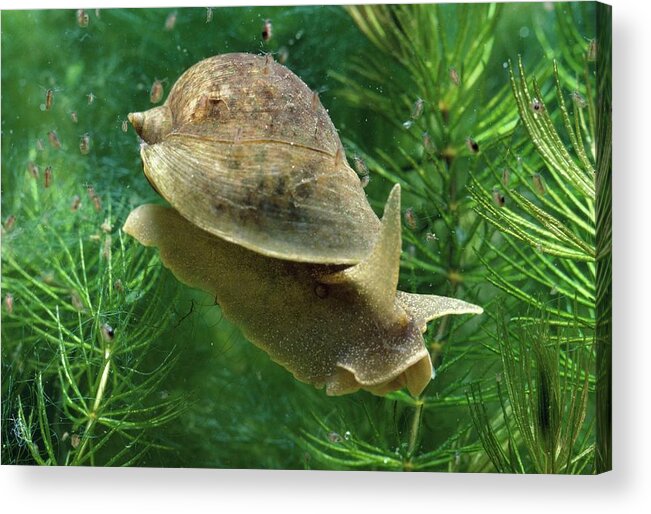A vivid, underwater photograph captures a gray snail with translucent horns against a backdrop of vibrant, green, fur-like aquatic plants. The snail, which closely resembles an apple snail, displays extreme detail, revealing the various parts of its body, shell, and possibly its eyes. It is suspended in the water, its worn, elegantly coiled shell suggesting it is not a juvenile. Surrounding the snail are numerous green fronds, creating a lush, healthy underwater scene. In the upper left, partially faded and indistinct, are other small creatures—potentially isopods or juvenile shrimp—adding to the dynamic environment. The bottom part of the photograph is slightly blurry, emphasizing the intricate focus on the snail and its immediate surroundings.